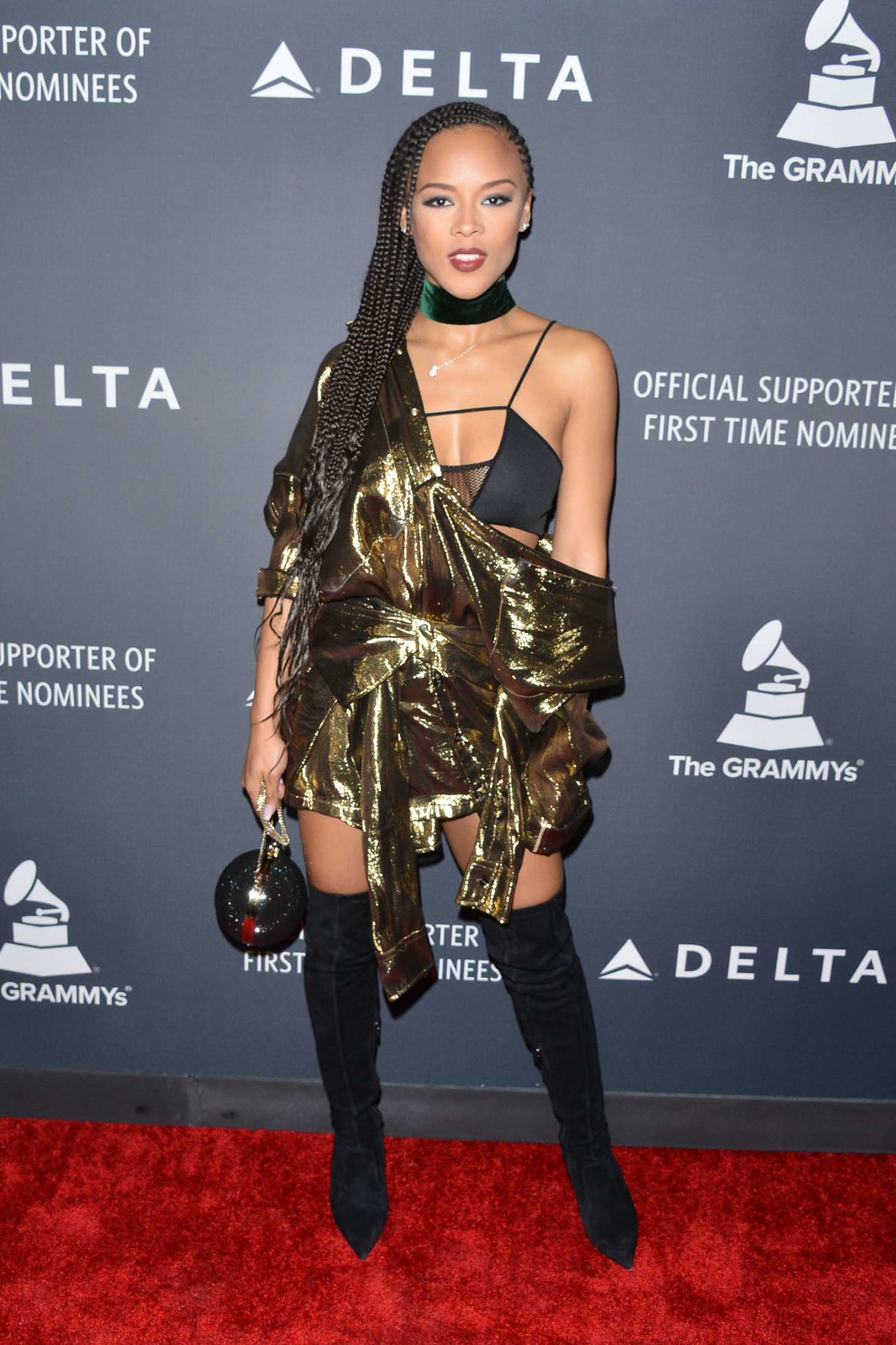At a red carpet event associated with the Grammy Awards, an African American woman stands out in a striking, meticulously put-together outfit. She is dressed in a gold one-piece ensemble consisting of coordinated shorts and a unique top. The top is designed with an over-the-shoulder style, revealing a delicate spaghetti strap tank top underneath. Towering thigh-high black boots complement her attire, and a chic velvet black neck wrap adorns her neck. Her long, braided hair cascades down, adding to her commanding presence. Behind her, a large banner features sponsors such as Delta and the Grammys, citing their role as the official supporters of first-time nominees, setting the glamorous backdrop for her standout appearance.